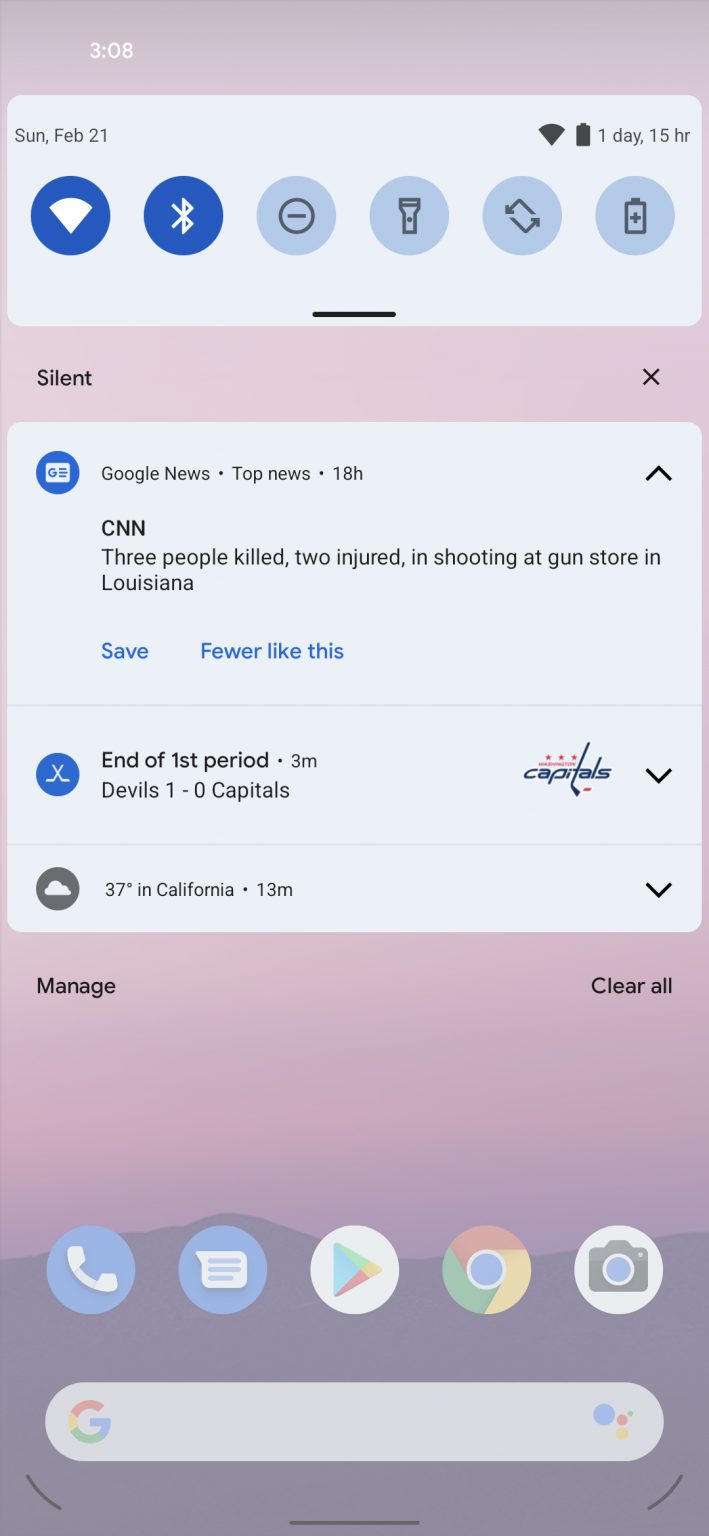The image showcases a smartphone screen filled with various notifications and essential details at the top and bottom. The prominent notification at the center is a CNN alert from Google News stating, "Three people killed, two injured in a shooting at a gun store in Louisiana." Just below that, there's a sports update indicating, "End of first period: Devils versus Capitals. Devils are winning." Further down, a weather notification displays, "37 degrees in California," likely in Celsius, which is notable given the usual use of Fahrenheit in the U.S. 

Above these notifications, a "silence" message is visible, suggesting someone has silenced notifications. The screen belongs to an unfamiliar phone model, potentially a Google device. The top of the screen shows the current time, Wi-Fi signal, and battery life indicator, with a battery estimate of a day and 15 hours remaining.

At the bottom of the screen, shortcuts for essential apps are visible, including Phone, Messaging, Google Chrome, and Google Play Store, along with a Camera icon. The date displayed on this typical yet informative smartphone screen is Sunday, February 21st.